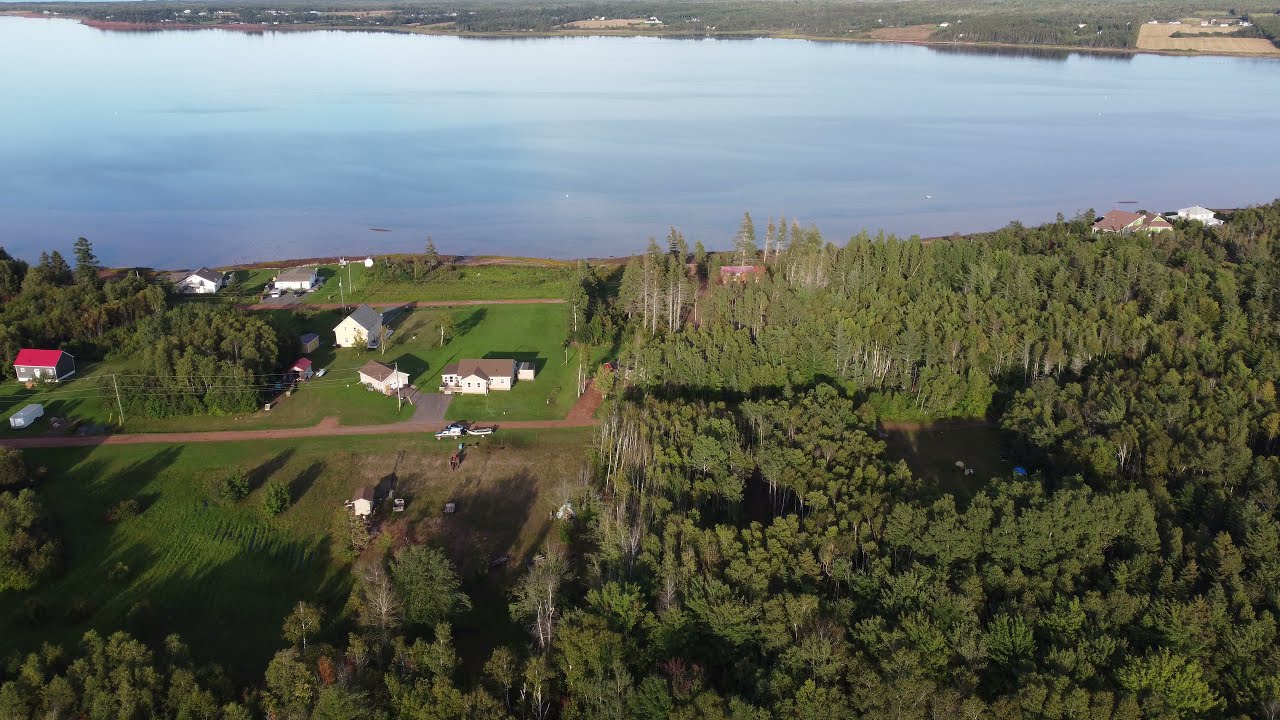This aerial photograph captures a picturesque, rural landscape featuring diverse elements. In the lower portion, a green expanse dominates, blending a densely wooded area on the right with a more open, farm-like property on the left. Tall, lush trees form a dense forest, contrasting with an assortment of residential buildings spread across the cleared land. Notable structures include several white houses, with one accompanied by a gray building with a red roof, and dirt roads crisscrossing the terrain. A car can be seen parked on one of these roads. The serene blue lake occupies the upper third of the image, reflecting a silver-blue hue, with the opposite shore lined by similar greenery and sparse structures. The tranquil water creates a natural border, bisected by rich foliage and scattered homes, encapsulating the serene, pastoral charm of the countryside.